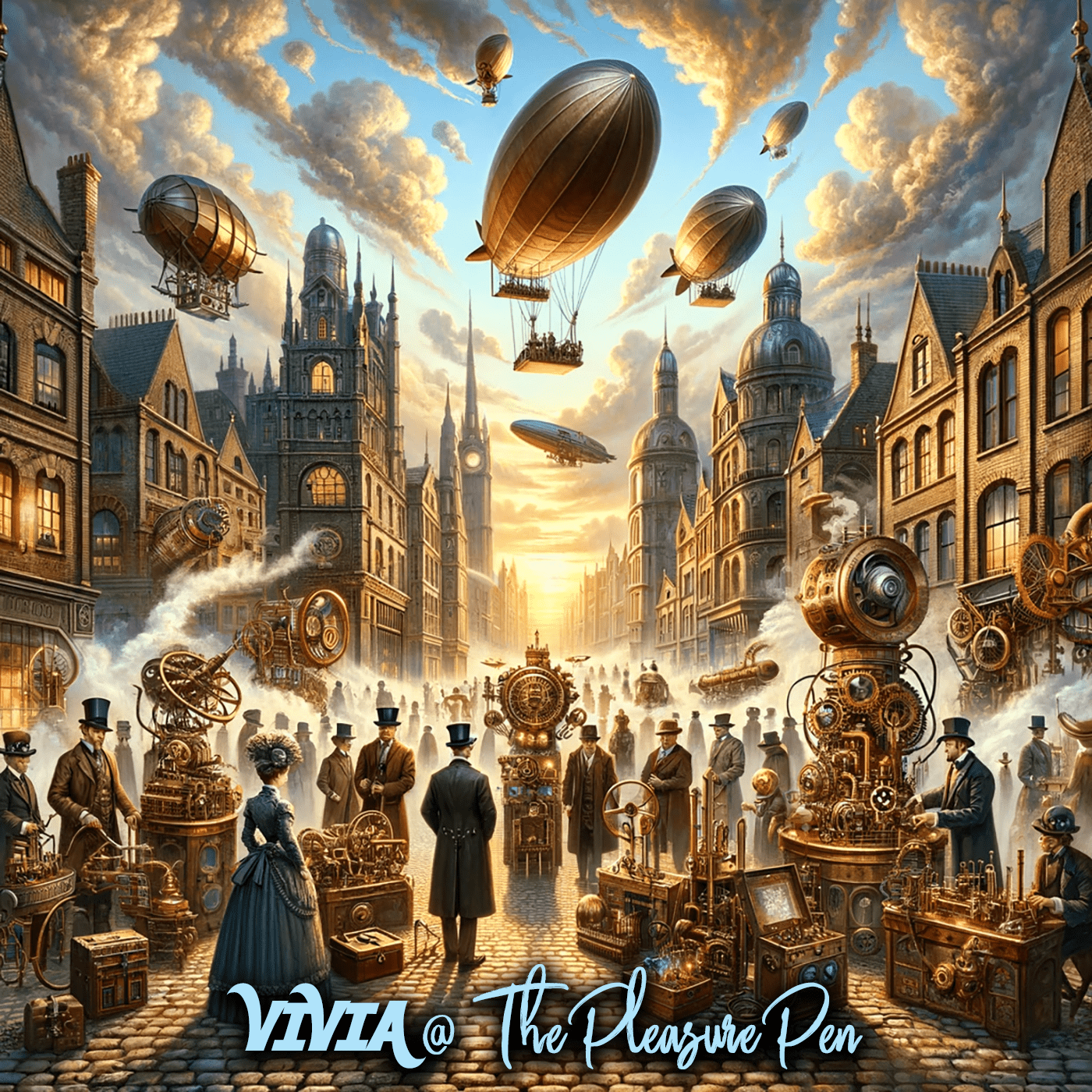The image is a steampunk-themed poster or advertisement, featuring the text "Vivia at the Pleasure Pin" in blue font at the bottom. It depicts a Victorian cityscape with a futuristic twist, showcasing tall brown and copper buildings with intricate spires and brick roads. The sky is a blue, cloudy expanse with a setting or rising sun, adding a dramatic ambiance. Several mechanical blimps, resembling hot-air balloons, float in the sky, each equipped with basket-like platforms carrying passengers. The streets are bustling with a crowd of people dressed in vintage attire; men in suits and top hats, and women in elaborate dresses. Among the crowd, there are various fantastical, golden-hued mechanical contraptions and inventions, exuding steam and enhancing the scene’s eclectic feel. Treasure chest-like objects and other ornate devices line the cobbled street, contributing to the busy, whimsical atmosphere of this steampunk world.